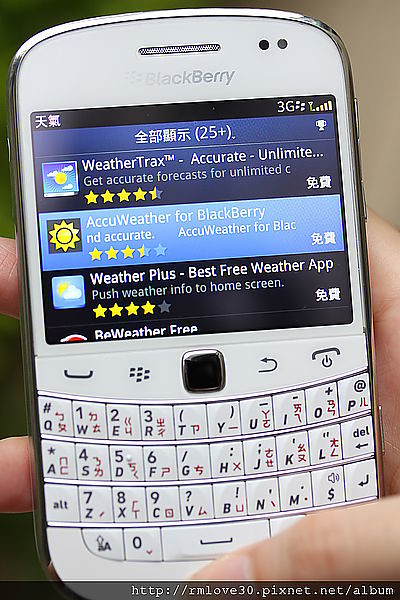This is a detailed close-up photo of an older model white BlackBerry smartphone, possibly a BlackBerry Bold. A light-skinned person is holding the phone with their right hand. The phone's top half features a square screen, while the lower half showcases a physical keyboard, both of which display Chinese characters, indicating it's a Chinese version of the BlackBerry. The screen, set in an app store, lists weather applications: "WeatherTracks Accurate" with four and a half stars, "AccuWeather for BlackBerry" with three and a half stars, and "WeatherPlus" with four stars. AccuWeather is highlighted. The phone runs on 3G technology, further dating this older model.